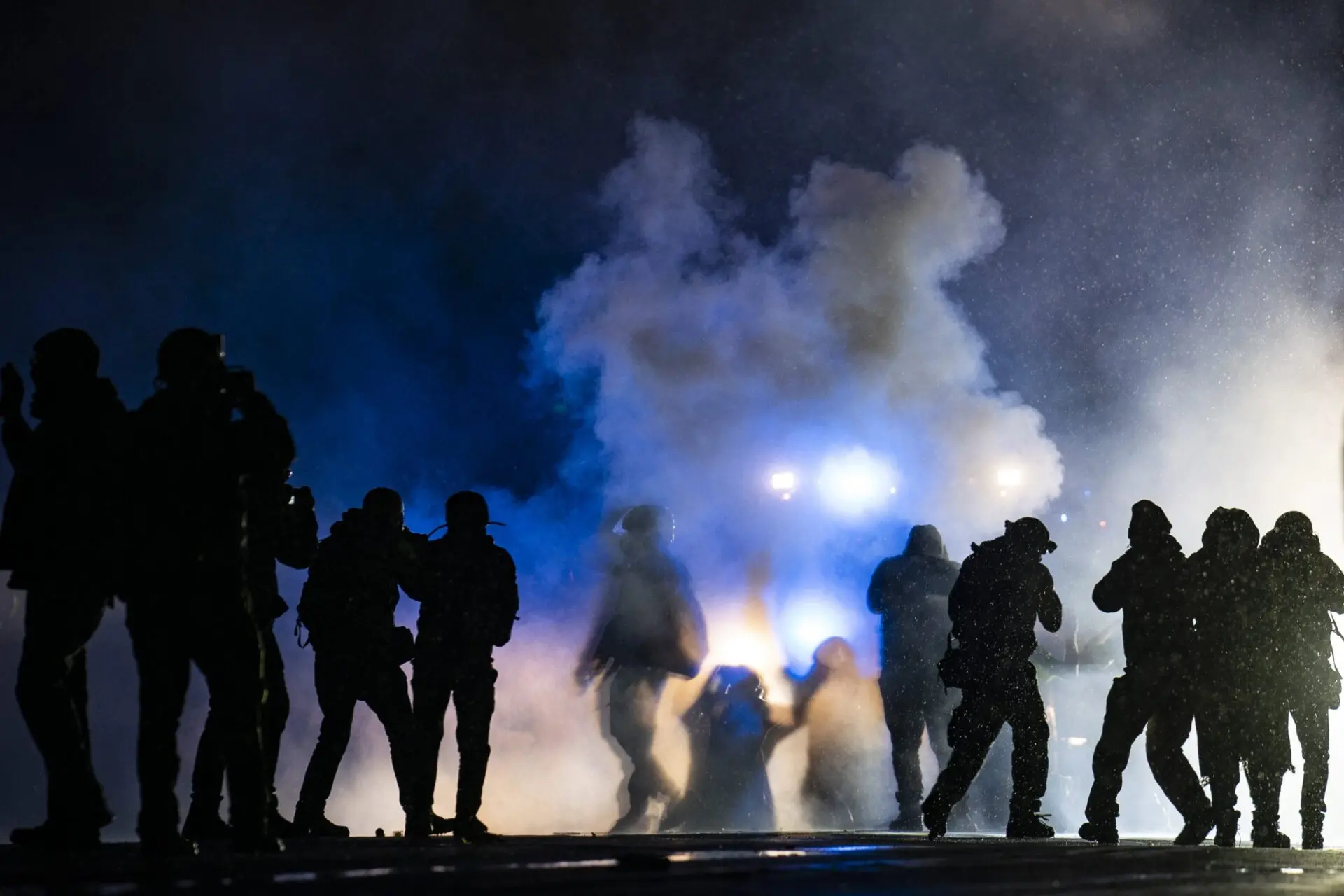In the midst of a dark, smoky night, an image captures a chaotic scene populated by shadowy figures, presumably firefighters, clad in dark uniforms. These figures, numbering approximately nine, are silhouetted by bright lights piercing through the dense smoke that blankets the area. The smoke, thicker and whiter in some areas and darker blue towards others, envelops the scene, creating a hazy atmosphere. One figure, discernible amidst the obscurity, appears to be kneeling. The ambient colors predominantly blend black, blue, white, and hints of yellow and orange, adding to the intense and dramatic feel of the night-time image. The overlapping presence of shadowy figures throughout the scene indicates a large group working amidst the smoky haze.